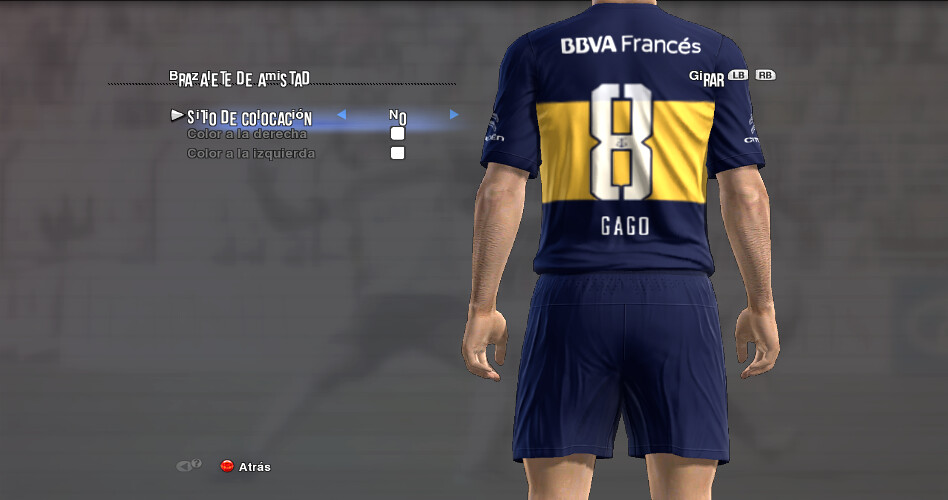The image depicts a video game character wearing a navy blue short-sleeved soccer jersey. The view is from below the neck to just above the knees, showcasing the back of the jersey prominently. The upper back of the jersey features the text "BBVA Francés" in white. Centered on the back is a large yellow rectangle with a blocky white number 8 inscribed within it. Just below the number, the name "GAGO" is displayed in white text. The character's shorts, which end above the knees, are also navy blue. To the top right of the character's body, a button indicator for "LBRB" is visible, suggesting in-game actions. On the left side, there are additional video game options in what appears to be Spanish, including "color a la derecha" and "color a la izquierda," indicating some customization features. The background is a plain, blurry gray, with no distinct features. This detailed depiction suggests it could be an advertisement or customization screen within a soccer video game, possibly similar to FIFA.